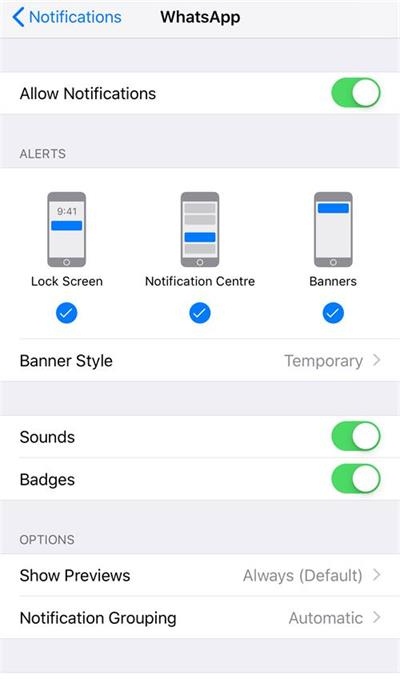The image depicts a smartphone screen with a notification settings interface for the WhatsApp application. The top part of the screen features a blue background with a blue box containing a left arrow and notifications in blue print, along with the word "WhatsApp" in black print. Below this, there is a blue box and a white box labeled "Allow Notifications" accompanied by a green toggle button. Following this is a blue button labeled "Alerts." 

Further down, a large white box is split into three sections:
1. "Lock Screen" with a blue dot and a checkmark.
2. "Notification Center" with a blue circle and a checkmark.
3. "Banners" with a blue circle and a checkmark.

Below this section is a small line, under which "Banner Style" with the setting "Temporary" followed by a right arrow is displayed.

Continuing down, there is another blue box, followed by two white boxes. The top white box is labeled "Sounds" and includes a green toggle switch. The second white box is labeled "Badges," also featuring a green toggle switch.

Next, there is a blue box labeled "Options," under which two more white boxes are present:
1. "Show Previews," set to "Always (Default)" with a right arrow.
2. "Notification Grouping," set to "Automatic" with a right arrow.

Finally, at the bottom of the screen, there is a blue box.